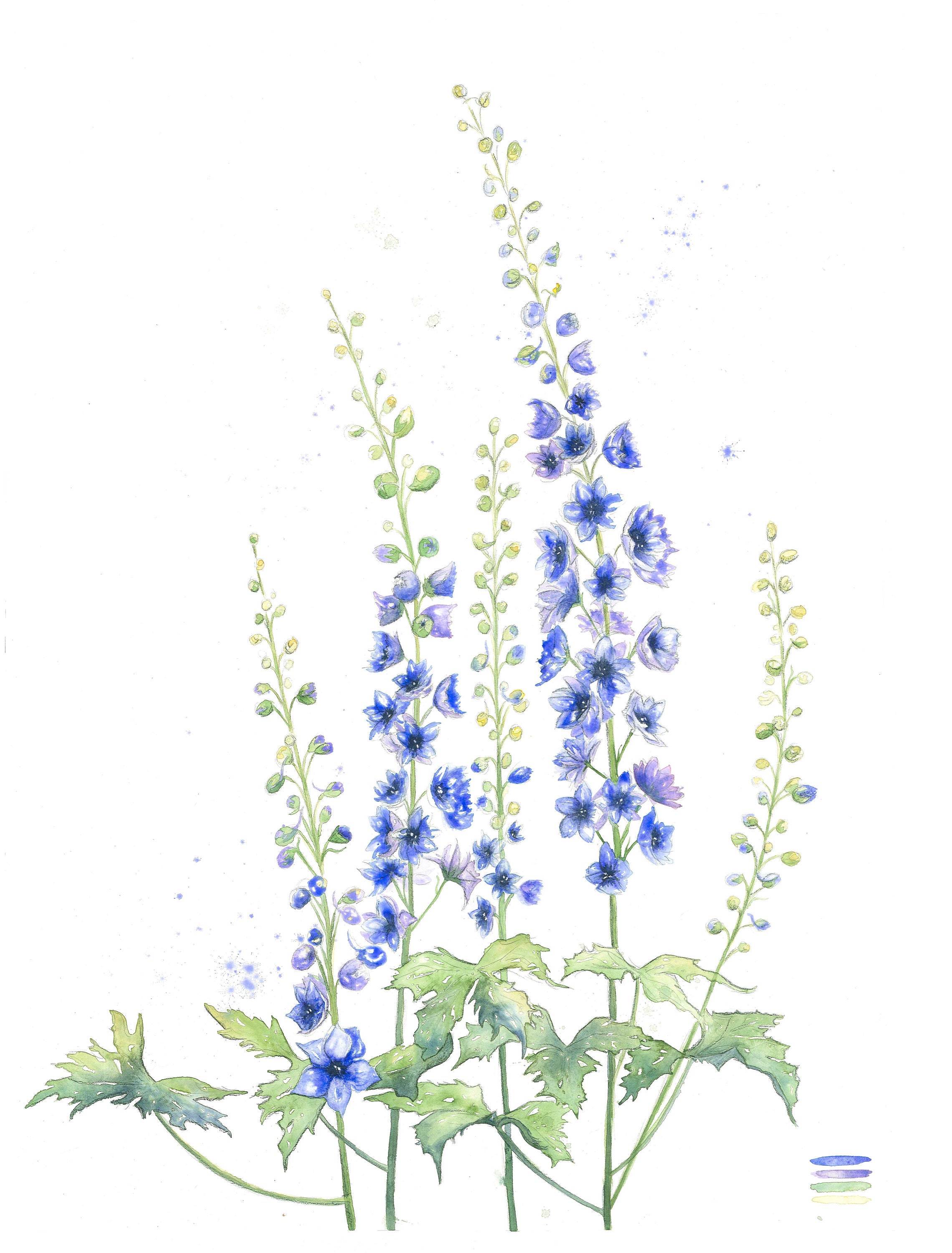This detailed illustration, set against a plain white background, showcases a delicate composition of four flower stems, each adorned with varying stages of blossoms and leaves. The stems ascend in a subtly curved but predominantly upright fashion, with the rightmost stem being the tallest. Each stem features light green leaves with irregular patterns and slight notches, adding a natural texture to the depiction. At the base of the image, there's evidence of color testing with faint stripes of yellow, green, purple, and blue, hinting at the artist's preparation and palette choices. 

The flowers themselves progress from budding to full bloom along the stems. The budding flowers exhibit hints of green and yellow transitioning into light purple, while the fully blossomed flowers are a rich blend of dark blue, purple, and subtle touches of white and pink. This variance captures the lifelike sequence of floral development. This meticulously painted scene, devoid of any distractions in the background, allows the observer to focus solely on the intricate details and vibrant hues of the flowers and their foliage.